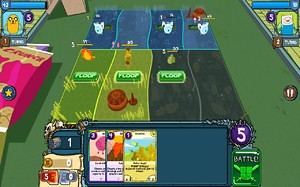A screenshot of a retro-styled, Adventure Time-themed game displayed on a computer monitor. The game features nostalgic, somewhat dated graphics reminiscent of early 2000s mobile or console games like those on the Nintendo Switch. It appears to be a fun, light-hearted party game rather than a competitive or hardcore title. In the top left corner, there's an icon of the yellow dog character, Jake, while the top right corner features the character Finn holding a golden sword. The main gameplay screen is divided into four fields, suggesting a versus-style card game format. At the bottom middle of the image, three cards are displayed within a grey rectangular frame. In the top right corner of this frame, a purple circle with the number '5' in white indicates an element of resource management, possibly representing elixir or playing power. Each player seems to have four thinner rectangles and a larger rectangle, likely used for defense or gameplay strategy.